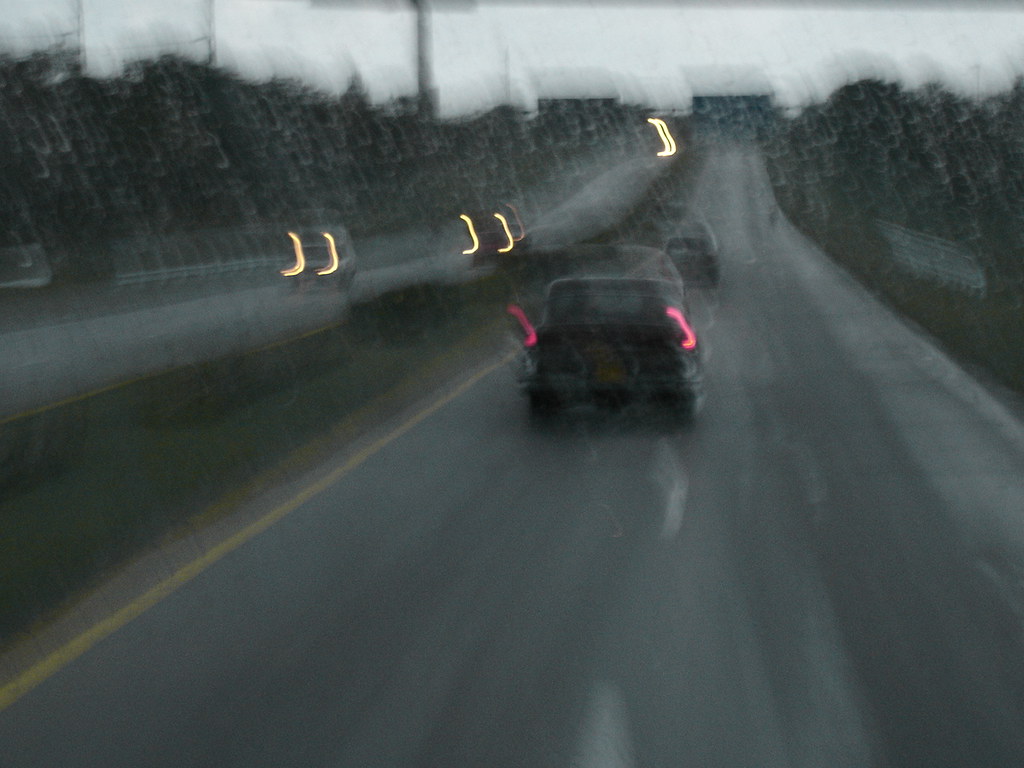This photograph captures the view from inside a car driving down a rainy, two-lane highway. The image is horizontally oriented and somewhat blurred, emphasizing the challenging visibility conditions. Through the streaked windshield, likely covered with rain droplets, we observe a red antique vehicle directly ahead and a black car with illuminated brake lights. On the left-hand side, the headlights of oncoming cars shine brightly, distorted by the rain and creating a shimmering effect. The overall atmosphere is overcast, with a gray sky looming above and trees faintly visible in the background. Road signs are present but unreadable due to the image's lack of focus, adding to the sense of obscured vision on this wet and dreary day.